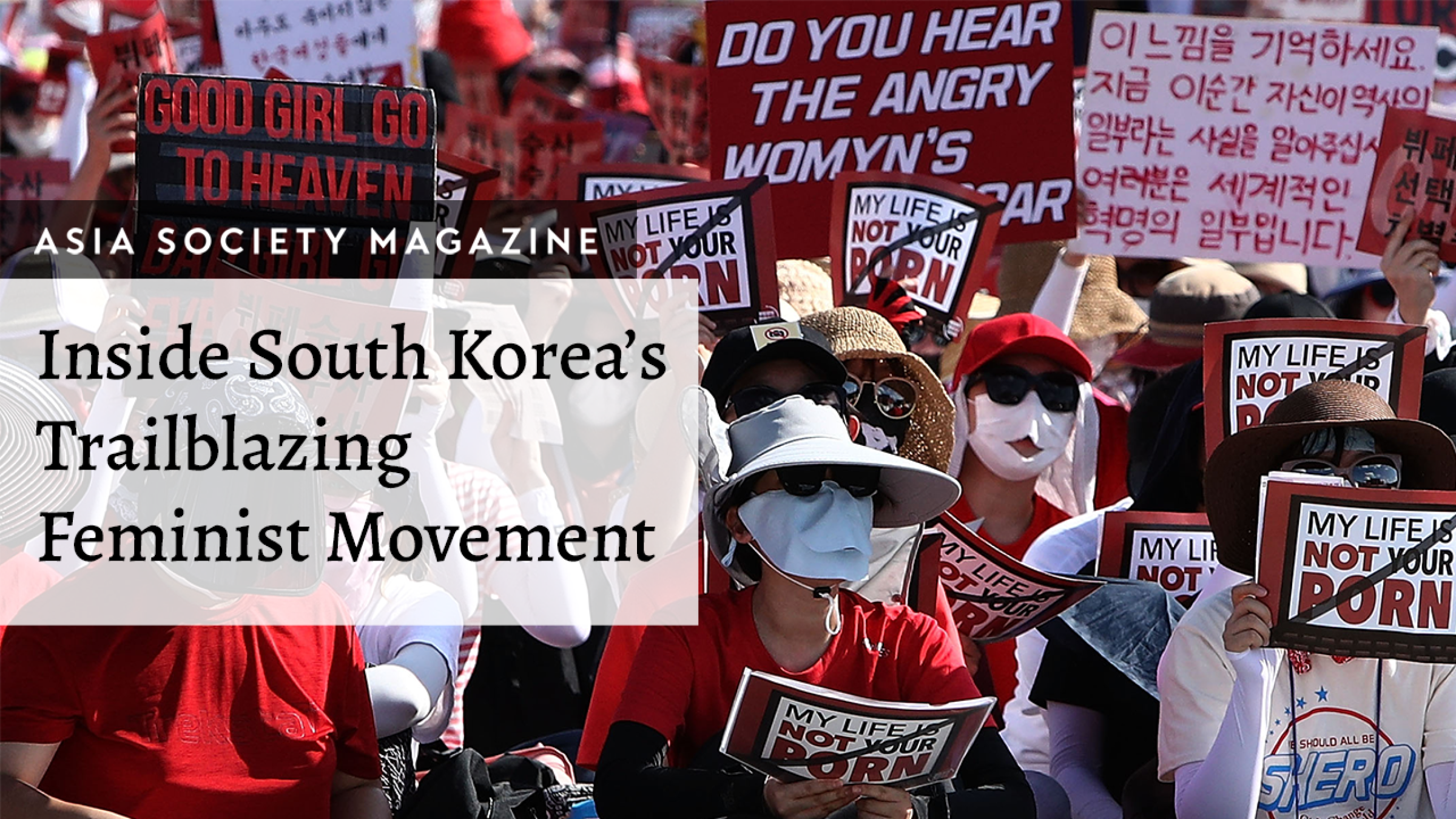This vibrant photograph, featured in Asia Society Magazine alongside the headline "Inside South Korea's Trailblazing Feminist Movement," captures a dynamic scene from a feminist protest in South Korea. The image prominently displays a diverse crowd of demonstrators, most of whom are women clad in various hats—ranging from red caps to straw hats—and all wearing face masks or scarves, which obscure their identities. A majority of the participants hold vivid red signs with bold black and white text declaring, "My life is not your porn." Other visible signs include messages such as "Good girl, go to heaven" and "Do you hear the angry women's roar?" with women spelled as "w-m-y-n." Additionally, one woman stands out in a white shirt emblazoned with "We should all be sheroes." While many of the protestors’ faces are partially obscured by their attire or the signs they hold, the determination and unity of the group are palpable. The backdrop reveals more partially blurred figures, capturing the scale and intensity of the daytime protest.